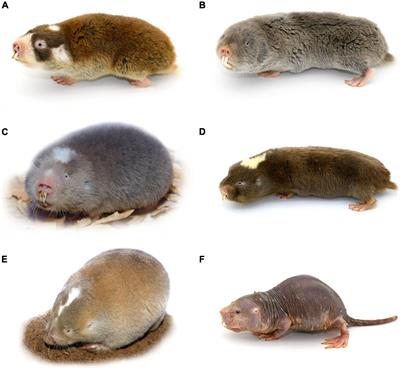The image displays six distinct rodent-like creatures, arranged in two columns of three rows each, labeled A to F. The top left rodent, labeled A, is small and brown with white detailing around the cheeks and snout. Its neighbor, B, on the top right, is thinner, gray in color, and looking towards the screen with visible large buck teeth. In the second row, C on the left is also gray but appears fatter with a white puff on top of its head and prominent teeth. D, to the right of C, is longer, thinner, and brown with a similar white puff, though its eyes are not visible. The bottom row features E on the left, a wider, fluffy rodent with light brown fur and a white stripe on its head, positioned on a brown surface. Finally, the bottom right showcases F, a gray, fur-less creature resembling a naked mole rat, with its eyes clearly visible. The background of the image is white, highlighting the distinct characteristics and textures of each rodent.